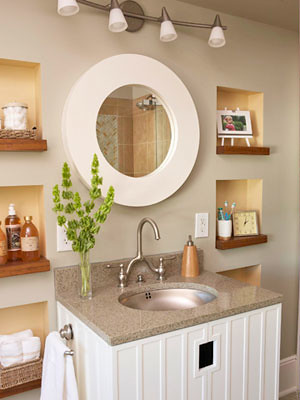This richly detailed photograph captures a country-style vanity within a beautifully designed bathroom area. The vanity, exuding a blend of integrated and freestanding characteristics, stands distinctively apart from other room elements. A highlight is its under-mounted basin that ensures water drips directly into the sink, paired with a sleek, two-handled faucet unified by a single arch spout.

To the left of the vanity, a lush green plant adds a refreshing touch, while a functional soap dispenser sits conveniently on the right. The design integrates practical elements, such as outlets on both sides, enhancing utility. A centerpiece of elegance, a circular mirror with a thick, off-white border hangs above the vanity, complemented by a sophisticated wall-mounted four-light fixture.

Surrounding the mirror, recessed areas feature shelves of a slightly darker hue, perfect for displaying perfumes, lotions, a clock, and even a charming picture of a dog atop a little easel. To the left, a towel hangs neatly on a rack, accompanied by additional washcloths stored in a wicker basket, adding to the country charm.

The vanity boasts a white front with a stunning brownish-gray speckled top, harmonizing with the adjoining walls covered in a unique reddish-gray hue. The entire arrangement flaunts a cohesive and delightful color scheme, embodying both style and practicality in this timeless, rustic bathroom design.